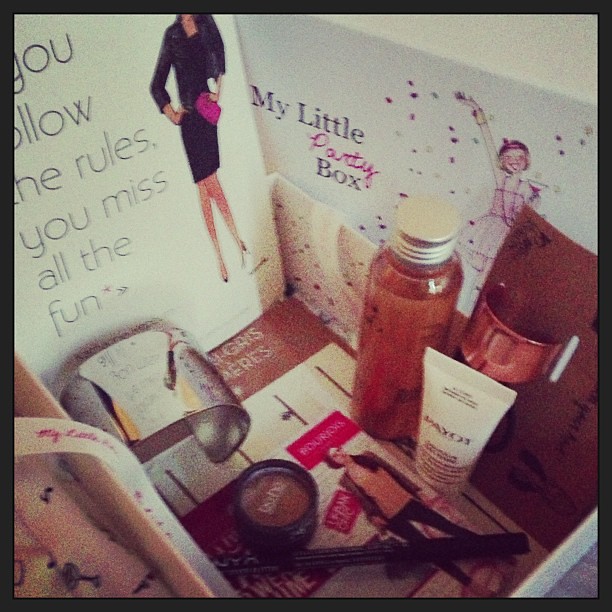The image showcases a detailed layout of items inside a themed "party box" designed for women. Prominently featured are two illustrated cards: one on the upper left bears the message "If you follow the rules, you miss all the fun" with a graphic of a woman holding a purse, while the other on the upper right reads "My little party box" and depicts a girl celebrating with confetti. The box is filled with various beauty products including makeup, jewelry, hair bands, and possibly a towel. Additionally, a fashion magazine and other feminine items are neatly arranged, some accompanied by ribbons and packaging materials. The party box, as highlighted by the cards, is a curated collection aimed at delivering a fun, stylish experience.